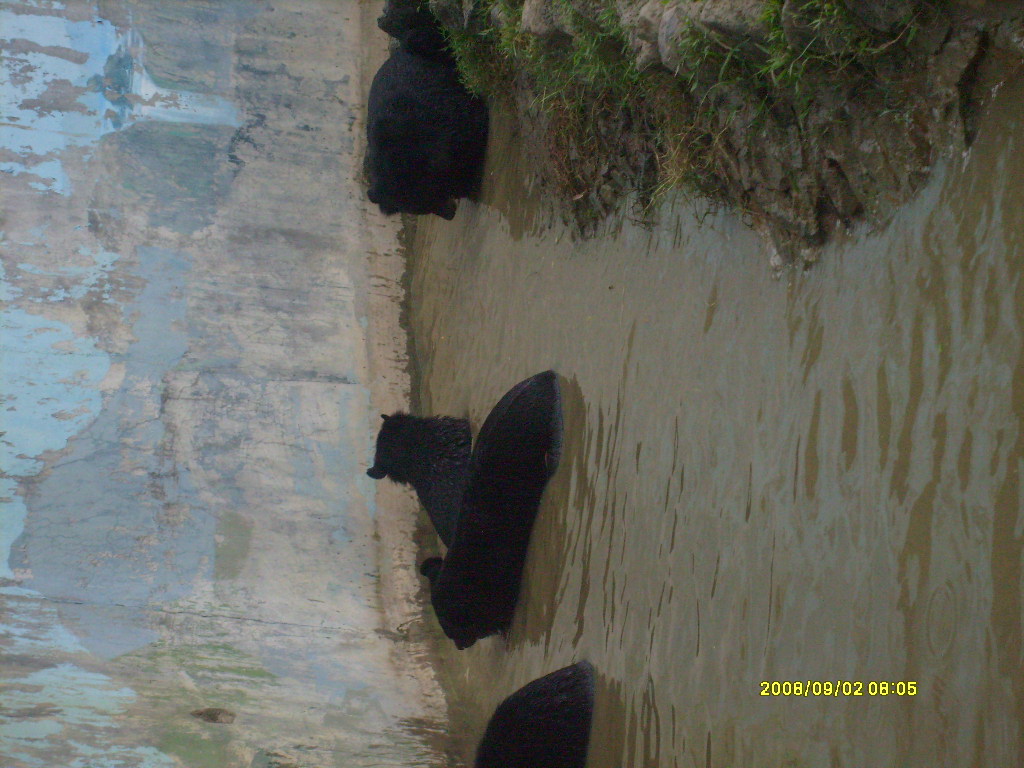The photo, taken sideways, captures a group of large black bears in an outdoor setting, possibly a zoo or wildlife refuge. They are seen in murky, muddy brown water amidst a muddy bank with sparse green grass on the right and a sheer rock wall to the left. Some of the bears are standing and walking, while others are lying in the water, with their broad, woolly backs and heads mostly turned away, except for one bear on the right. A peeling blue wall with exposed colors is visible on the left side of the image. A yellow timestamp reading "2008/09/02 08:05" is positioned in the bottom right corner of the photo.